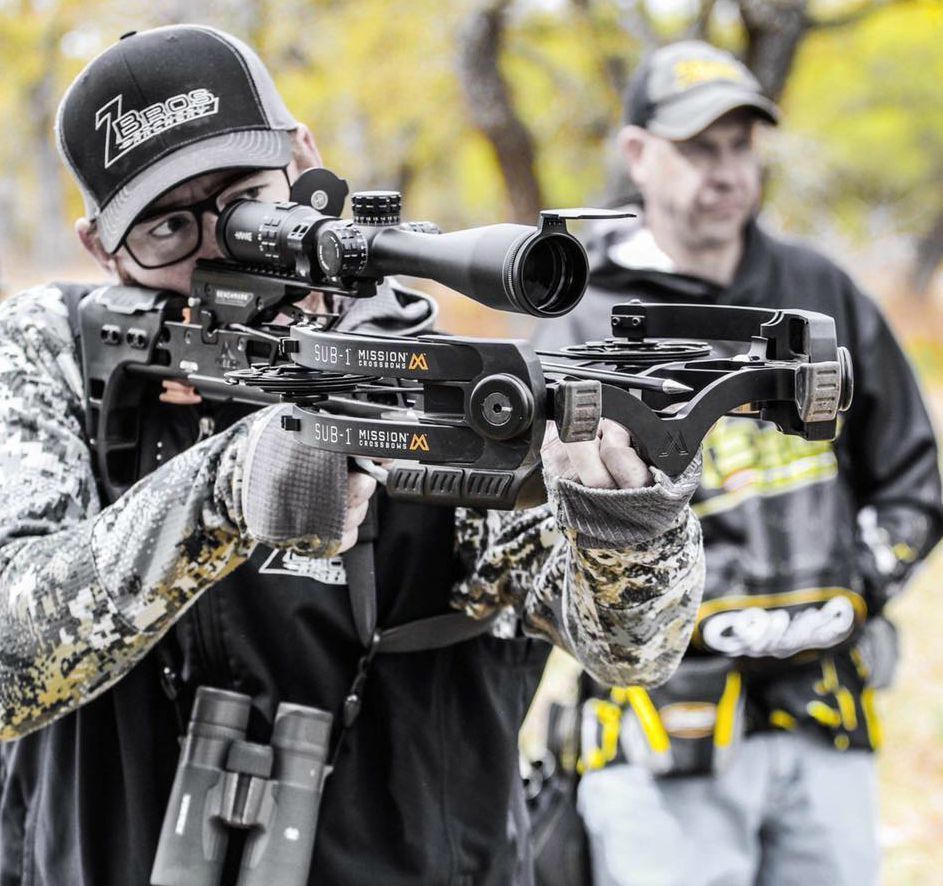A detailed close-up image captures two men dressed in black, white, gray, and yellow camouflage attire. The men, both wearing long-sleeved camo shirts and black vests, also sport camouflage-patterned pants and baseball caps. The man on the left, prominently featured in the foreground, wears black glasses and a black cap with a white zebra's archery logo. He is intently aiming a black crossbow labeled "Sub-1 Mission," bracing it against his chest while looking through the scope. Additionally, binoculars hang around his neck. The man on the right appears further back and is slightly blurred. The background reveals an outdoor setting with indistinct, blurred-out trees, emphasizing the focus on the man and his crossbow.